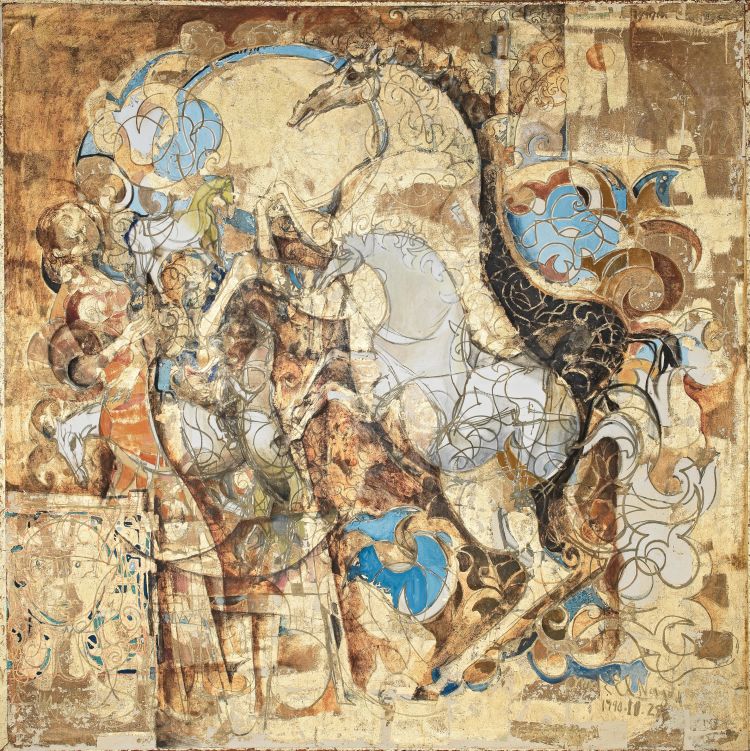This abstract artwork features a collage-like arrangement with a predominant background of various shades of brown, creating a textured and pieced-together appearance. At the very center, a thin silver horse rears up on its hind legs, with its face notably slim and accompanied by darker gray swirls near its lower body. Surrounding this central figure are multiple other horse outlines, including a yellowish horse rearing up above the silver one, and a smaller gray horse to the left. Additionally, there is a greenish and gray horse with a partially downturned head pointing to the left. The image includes splashes of blue, tan, black, and white hues. On the left side, there are several rotated human figures in various orientations, adding to the artwork’s complexity. The entire piece, possibly a watercolor or pencil drawing, is accented with wavy lines and a blurred, almost dreamlike quality.